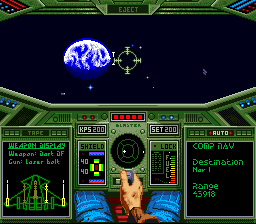Screenshot from a vintage video game: The image depicts a player character seated in the cockpit of a starcraft, gazing out through a large window into the vastness of space. The Earth is visible in the distance, partially obscured in shadow yet displaying its characteristic blue and white swirls. The cockpit interior is a dark green, adorned with numerous panels, buttons, and sensor readings. The protagonist, dressed in a red long-sleeved coat, extends their hand towards a joystick, likely used for navigating the ship. To the right, a navigation panel labeled "COMP NAV NAV" is shown, indicating an active destination. On the left, another panel displays the schematics of the ship, providing critical system information to the player.